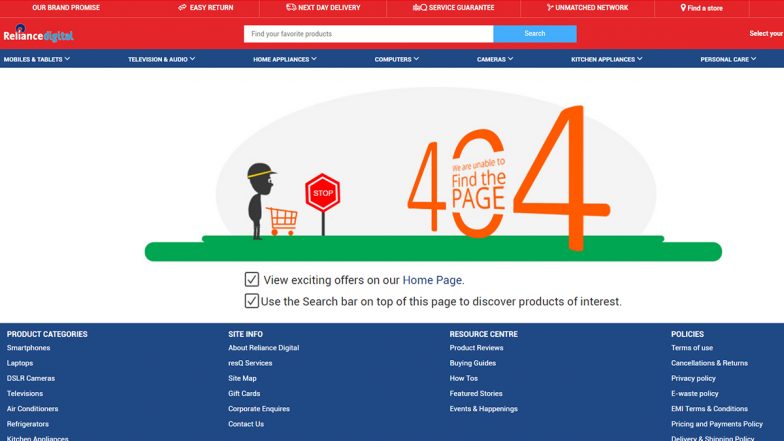In this image, the top left corner prominently displays the website name "Reliance Digital." To the right of that, centrally positioned, is a search bar with the placeholder text "Find your favorite products," accompanied by a blue rectangular search button labeled "Search" on its right. Just below this, a horizontal menu presents various categories in a sequence: "Mobiles and Tablets," "Television and Audio," "Home Appliances," "Computers," "Cameras," "Kitchen Appliances," and "Personal Care," with each category name in white text on a blue background.

In the middle section of the image, there is a 404 error message highlighted in orange, indicating a page not found. Next to this message, on the left, an illustration features a person with an orange shopping cart sitting in front of a red stop sign.

Below this, two checked square boxes with corresponding text appear. The first box has a message to its right, stating "View exciting offers on our home page," with "home page" highlighted in light blue. The second box has the text "Use the search bar at the top of this page to discover products of interest."

Finally, at the very bottom of the image, there is a section with a dark blue background, showcasing links to various categories: "Product Categories," "Site Info," "Resource Center," and "Policies."